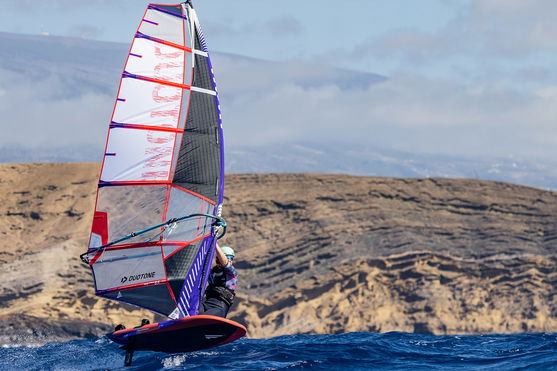In this image, we see a dynamic scene of windsurfing against a striking natural backdrop. The main subject is a person engaging in windsurfing on a choppy, vibrant blue ocean, their board seemingly skimming just above the water's surface. The windsurfer is outfitted in a sleek black wetsuit, accented by a blue vest and a protective white helmet. They are tightly gripping the mast of a visually striking sail.

The sail features a complex, geometric design composed of bold colors — primarily red, white, blue, and gray. Notably, the sail includes patches that are somewhat transparent, allowing glimpses of the rocky, rugged hills behind it. These hills have a diverse palette of earthy tones, including tan, brown, and specks of black. The hills extend across the entire width of the image, guiding the viewer’s eye toward a more distant mountain range shrouded in a veil of misty clouds.

Further enhancing the dramatic setting is the sky, a partly cloudy expanse with thin streaks of gray clouds interspersed with patches of pale blue. The overall atmosphere suggests a windy day, perfectly aligning with the action of windsurfing. The ocean water, characterized by its rich, dark blue hues, contrasts beautifully with the light and texture of the landscape. The scene captures the excitement and motion of the sport, set against an awe-inspiring natural environment.